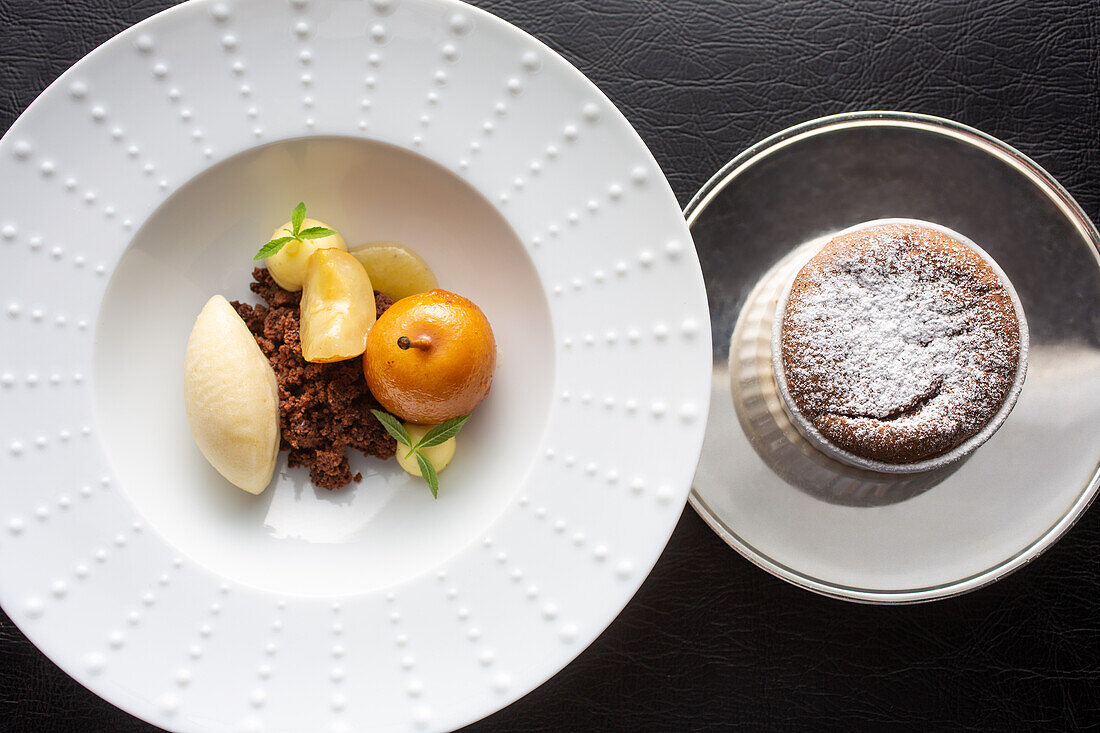The image features a photograph taken from directly above, capturing a sophisticated culinary presentation. On the left side of the image, there's a distinctive white bowl-plate hybrid with an intricate small round design on the thick border. The indented central area of this dish contains a modest portion of food, including slices of fruit—possibly apples or melon—strategically arranged alongside what appears to be meat. Notably, there are elements like an orange-hued fruit with a stem and round pieces with green fig leaves for garnish, adding an aesthetic touch.

On the right side of the image, there's a glass plate that slightly overlaps with the left dish. Centered on this plate is a small white dish, likely a souffle cup, filled with a chocolate-colored dessert sprinkled with powdered sugar. The background setting for this elaborate display is a stark black surface, possibly a countertop, highlighting the elegance and refinement of the dishes, suggesting a high-end dining experience.